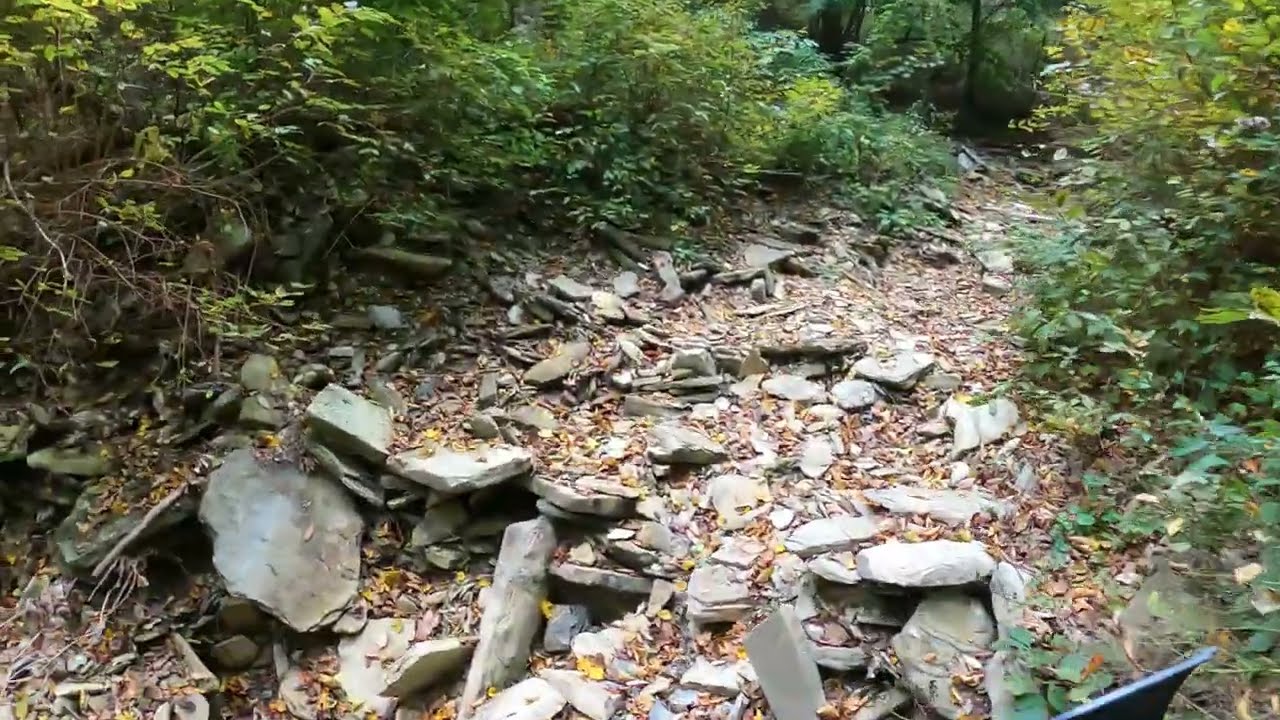The photograph depicts a rugged forest trail, likely deep within a wooded area. Dominating the center of the image is a path cluttered with jagged, gray rocks interspersed with dead leaves, suggesting a mixture of natural and possibly man-made elements. The trail, filled with these flat stones, appears challenging to navigate. Green foliage, including bushes and weeds, flanks both sides of the path, creating a dense thicket of vegetation. One notable small tree trunk is visible in the background, reinforcing the woodland setting. The trail expands wider at the bottom of the image and narrows as it extends to the top right. The scene indicates late summer or early summer, given the light green hue of the leaves. There are no people or text present in the picture, providing a solitary and untouched feel to the natural environment.